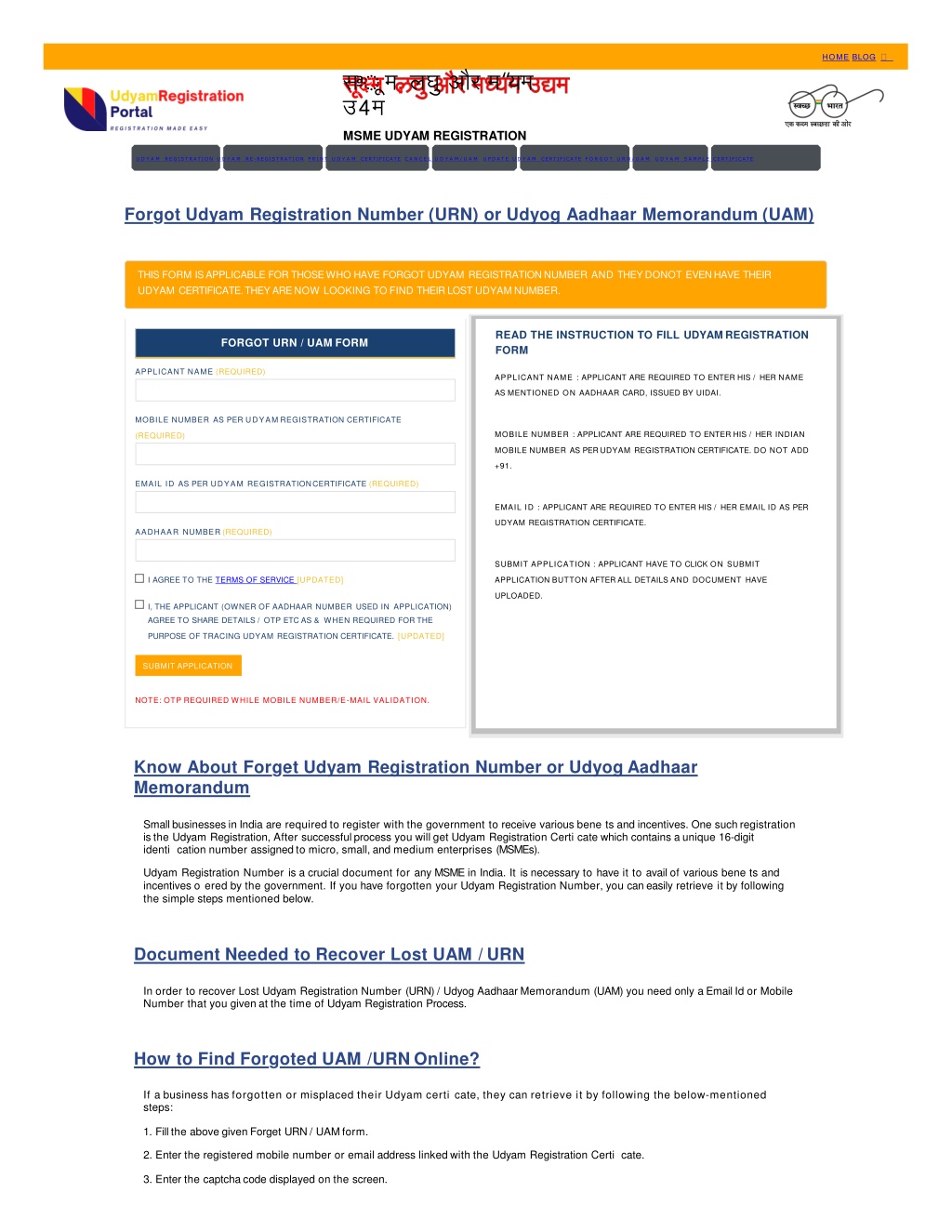The image depicts a section of the YADYAM Registration Portal. The title "YADYAM" is prominently displayed in yellow, with "Registrations" written in red, both set against a blue background. Below this title, there is a section containing text in an unidentified foreign language, possibly Arabic or an Asian script, surrounded by various colorful elements.

At the top of the portal, an orange bar runs horizontally from left to right, and to its right is a small emblem resembling a spectaсle, with additional text in another foreign language.

In the central part of the portal, the text "MSME YADYAM Registration" is displayed, accompanied by several grey buttons, some of which are difficult to read due to the dark blue text on a grey background. There are a total of seven grey buttons.

Further down, there's a section titled "Forgot YADYAM Registration or Adaga Adhar Memorandum," followed by a form intended for users who have forgotten their YADYAM registration number. Instructions to fill out the YADYAM registration form are provided, requiring details such as name, mobile number, and email ID. Links are available for users to access more information on recovering forgotten registration numbers.